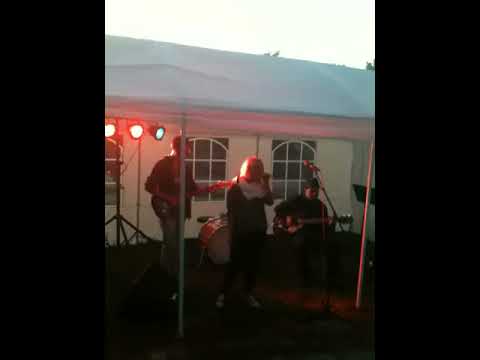The image captures a three-piece band performing under a white canopy, commonly used for outdoor events like weddings. From left to right, the band consists of a man playing a black guitar, dressed in a black jacket and blue jeans, standing under the warm glow of several lights. In the center stands a blonde woman, the lead singer, who is gripping a microphone close to her mouth. She is adorned with a white scarf around her neck and dressed in dark clothing. Behind her, a drum set with a kick drum, cymbal, and stool is visible, though no drummer is present. On the far right, a man with darker skin, possibly of Indian descent, is seated and playing either a guitar or bass, also dressed in dark clothing and possibly wearing a hat. The scene is set against the backdrop of a building with at least three large windows, under an overcast sky. The entire scene gives an intimate vibe, suggesting a small, private performance. The photograph focuses solely on the band, surrounded by various musical equipment and dimmed strobe lights, without showing any audience.